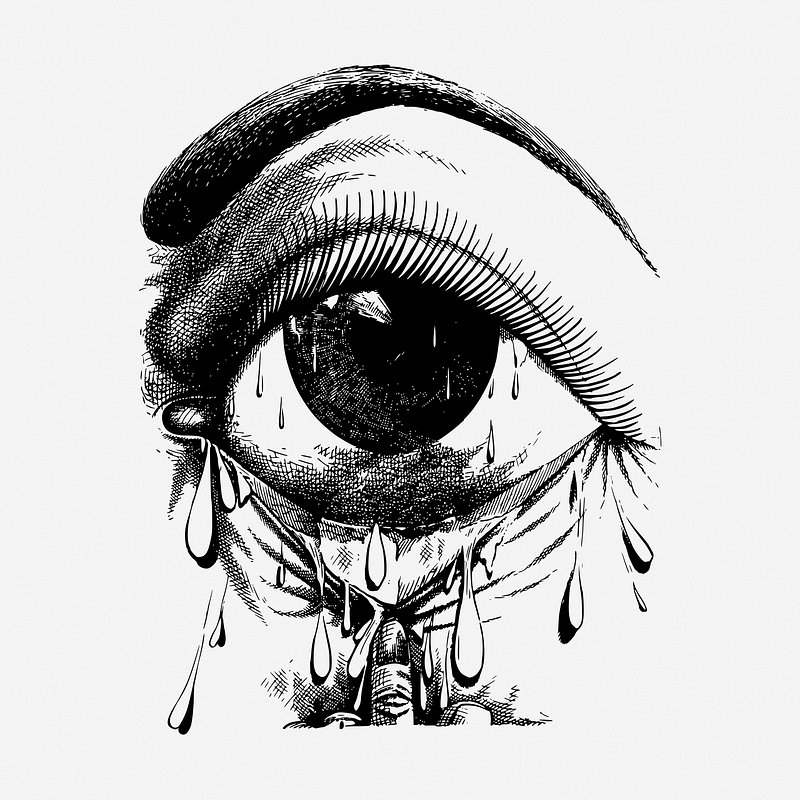The black-and-white illustration vividly portrays a close-up view of a single, weepy left eye. The eye is depicted with a large pupil and iris, with intricate shading and reflections to highlight its depth. A dark, well-defined eyebrow arches above the eye, contributing to the overall expressive mood. The eye's eyelashes are evenly spaced, adding to the drawing's detailed realism. An undersized finger with a dark fingernail is seen pulling down the lower eyelid, exposing more of the eye's white. Numerous tears are illustrated, with large, cartoonishly oversized drops cascading from both the upper and lower eyelids. The background remains stark white, making the meticulously drawn elements of the eye, including the shadows and creases, stand out prominently.